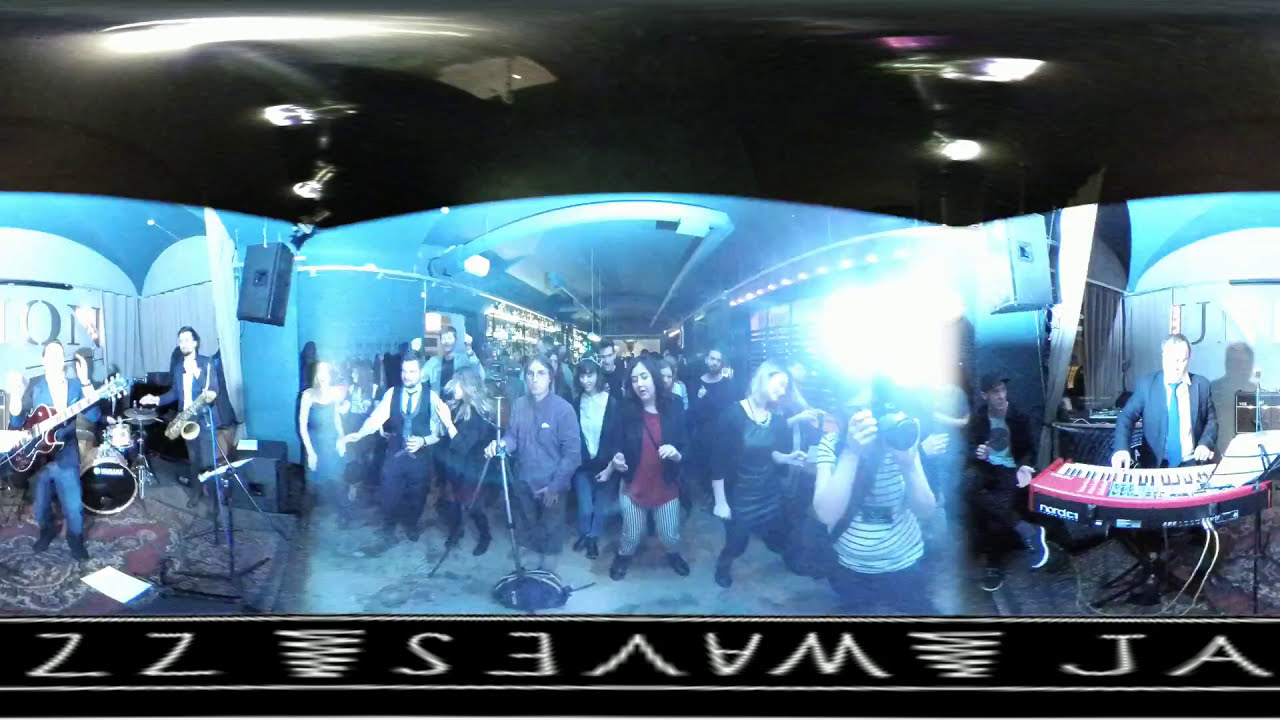This detailed panoramic 360-degree image captures the lively atmosphere of a music club concert, featuring a bustling bar scene and a dynamic on-stage performance. The stage section, due to the panoramic effect, appears split with the continuation of the same band members on both the right and left edges of the image. On the left side, there's a guitarist, possibly also the singer, clapping and playing the guitar, and behind him, a drummer playing on a Yamaha drum set. A saxophonist is also visible on this side. The band's faces are somewhat washed out due to the bright stage lights. The right side of the image highlights a close-up of the red keyboard, with a man intensely playing, surrounded by sheet music and wires.

In the center of the image, you see a crowded audience area where people are enthusiastically standing and dancing to the music, dressed in various colorful attire suggesting a vibrant, festive event. A striking flash can be seen from a camera within the crowd, illuminating part of the scene. Towards the back of the audience area, shelves possibly stocked with glasses hint at a bar setting, enhancing the club ambiance. The overall tone of the image is suffused with different shades of blue, attributed to a filter applied during the capture. The ceiling, painted black with recessed lighting, adds to the club’s intimate atmosphere.

At the bottom of the image, there is a superimposed graphic of distorted letters and symbols stretching across the scene. It reads "ZZ WAVES JA," with some letters upside down and backward, adding a layer of visual intrigue to the photograph.